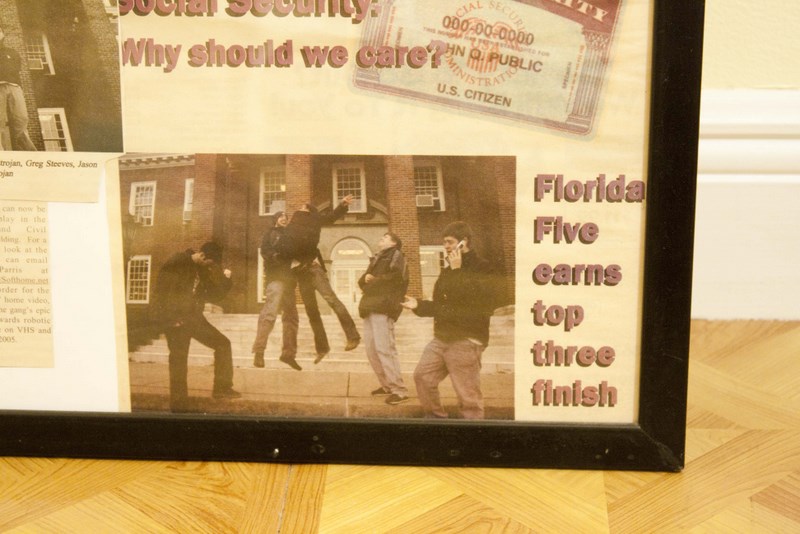A framed, commemorative newspaper clipping sits propped against a white wall on a light wood floor, its black frame visible only at the bottom right. The image inside the frame is faded with a yellowish tinge, showing signs of sun damage. Central to the clipping is a photograph capturing a lively scene where five young men, all wearing winter jackets and pants, energetically interact. Two of them are caught mid-air, seemingly engaged in a chest bump, while another holds a cell phone to his ear, laughing. These men stand in front of a brick academic building, distinguished by its multiple windows and arched entrance. Adjacent to this image, a caption reads "Florida Five earns top three finish." Above the photograph, there's an enlarged image of a Social Security card bearing the name "John Q. Public" and the number "000-00-0000," accompanied by the question, "why should we care," partially cut off at the top. The bottom molding along the baseboard is visible behind the frame, adding to the setting's homey feel.